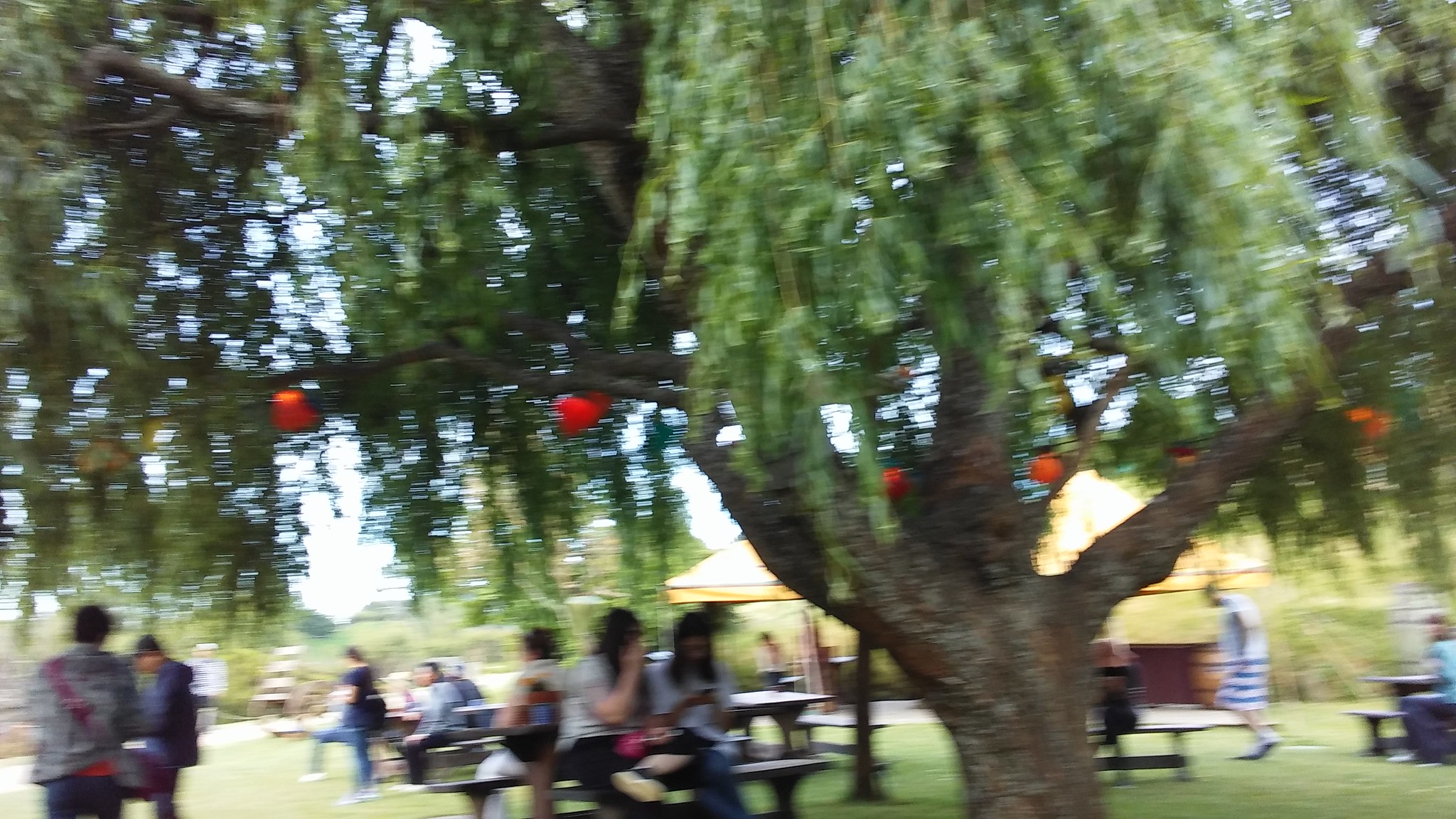A slightly out-of-focus photograph captures an outdoor scene dominated by a large, shaggy tree in the foreground. The tree, with its thick trunk and vertically hanging branches, creates a striking focal point. Attached to its branches are numerous red balls, possibly lights, adding a festive touch to the natural setting. Underneath the tree, people are seen milling about, some seated at picnic benches while others are walking nearby. In the background, a building is partially visible, completing the serene outdoor ambiance.